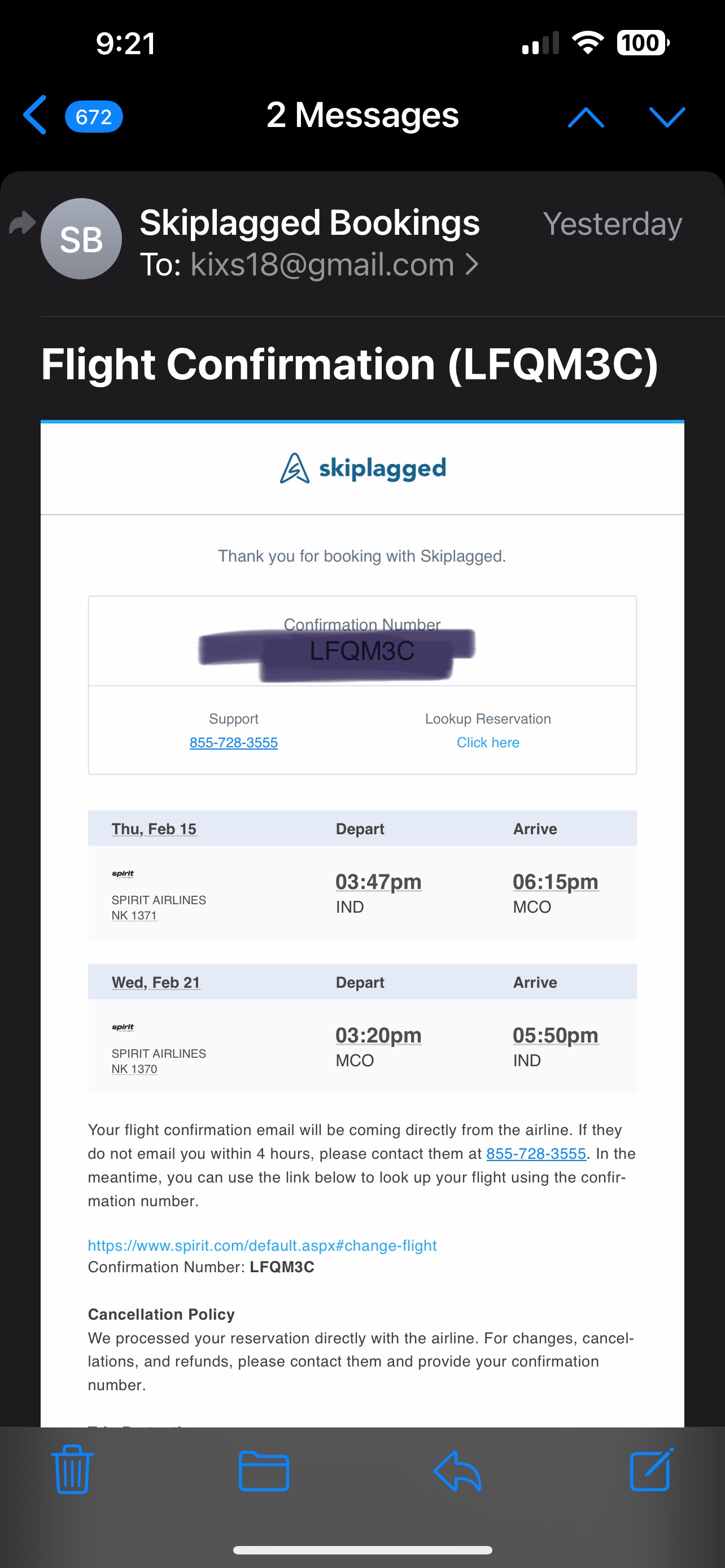This screenshot, taken from a smartphone with a black background, displays a message from the travel site SkipLagged. The phone's status bar shows it's 9:21 AM, with two bars of cellular signal, Wi-Fi connected, and a fully charged battery at 100%. The prominent white-centered message, which is part of a series from 'SkipLagged Bookings,' was received yesterday and is addressed to TIX18@gmail.com. It details flight confirmation LFQM3C. The SkipLagged logo, a minimalist triangle, sits to the left of the brand name. Below the logo, a thank you note reads, "Thank you for booking with SkipLagged." The confirmation number LFQM3C is repeated but obscured by a black highlighter. The itinerary includes a flight departing on Thursday, February 15th and returning on Wednesday, February 21st.